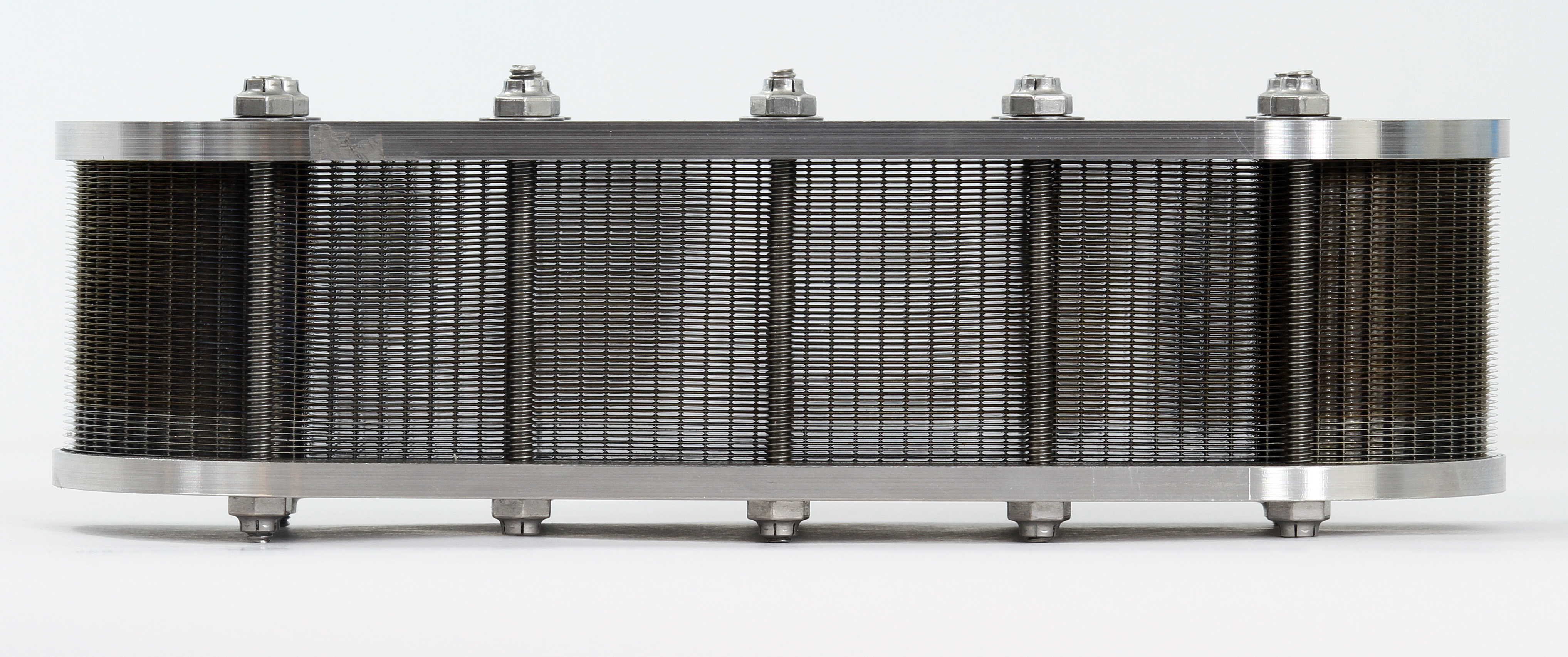The image depicts a large, silver metallic object, approximately two feet long and six inches high, resembling a metal screen or filter typically used in machinery or air conditioning units. This object is constructed from two thick steel plates with a grainy mesh screen in between, creating a "metal sandwich" effect. The mesh screen slightly curves around the edges and allows for partial visibility of the internal components. Five heavy, silver bolts threaded with nuts secure the steel plates together. These bolts are equidistantly spaced, with one centrally located and two more on each side. Notably, four of these bolts have their rough ends pointing upwards, while one bolt's end points downward. The overall structure has clean, black ends with a gray and clear middle section, giving it a polished appearance. The assembly seems to integrate both aesthetic and functional elements, indicative of a sophisticated piece of machinery or equipment.